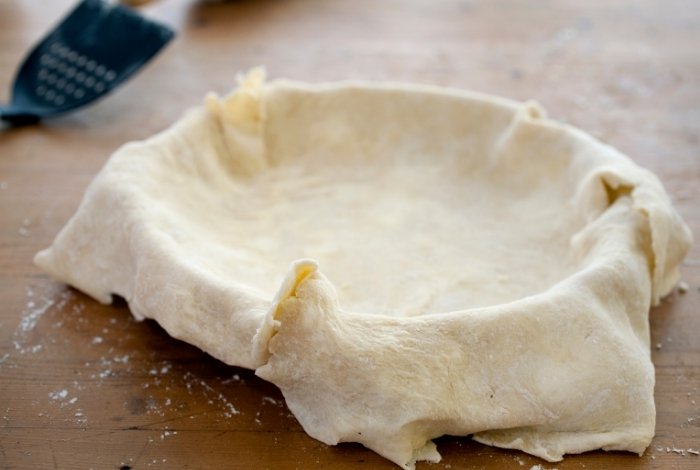The photograph captures an unbaked, white pastry crust draped over a circular pie dish, entirely covering the dish itself. This dish is placed on a flat, brown wooden surface that is dusted with specks and crumbs of flour and pastry, suggesting a busy kitchen environment. The crust appears to have been freshly rolled out and is hanging over the edges of the pie dish, ready to be shaped and filled, likely to become a delicious pie. In the top-left corner of the image, a black spatula with multiple perforations is partially visible, with its handle extending out of the frame. The setting exudes a homely and rustic preparation scene, as if someone is in the midst of a baking project, surrounded by the simple tools and floury mess typical of such culinary endeavors.